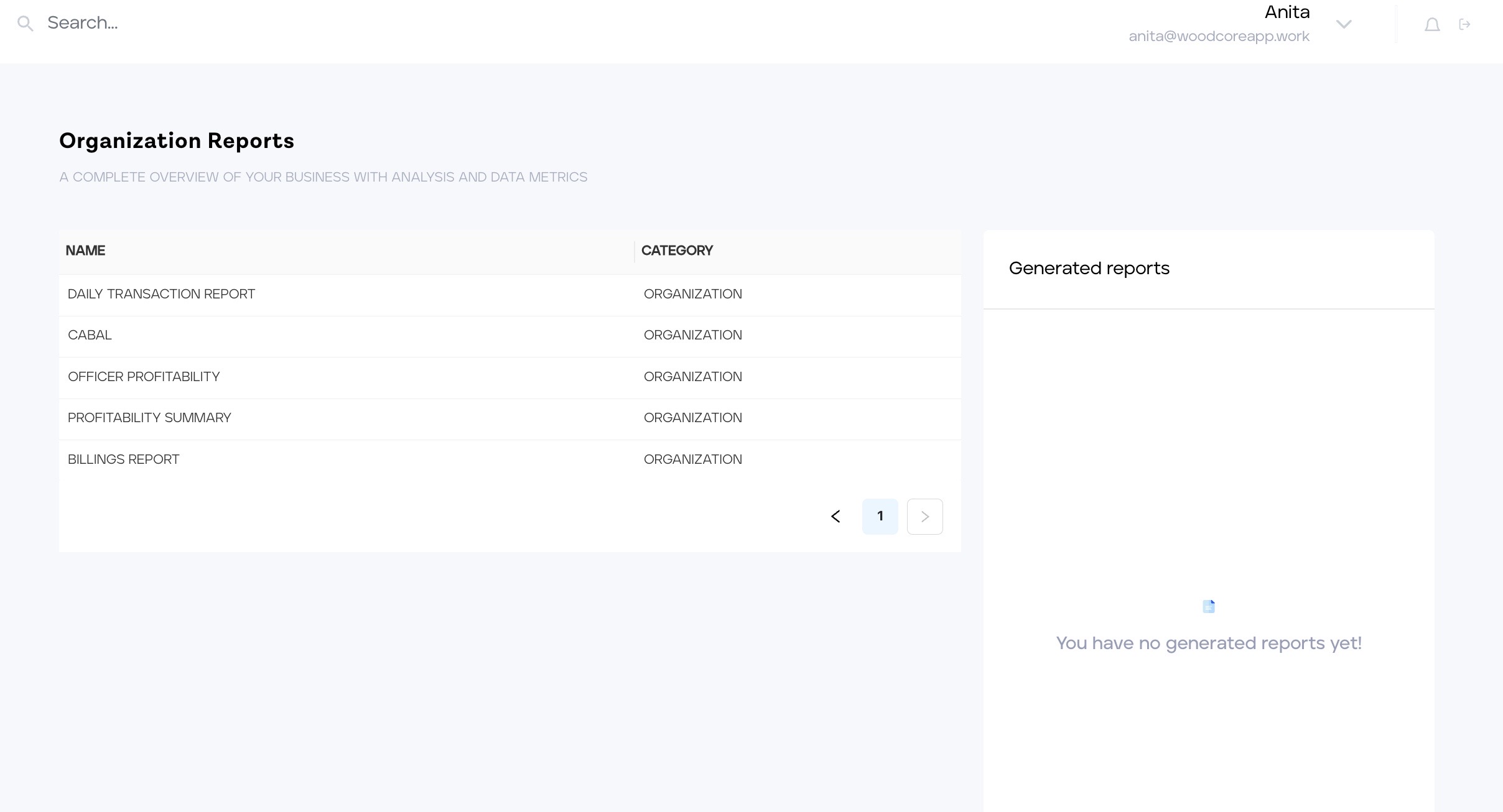The image features a sophisticated user interface on a white background. At the top, there is a gray magnifying glass icon accompanied by the word "Search" in gray font. To the right of this, the name "Anita" appears next to a downward-pointing gray arrow. Below this section, the email address "Anita@woodcrep.work" is displayed, followed by a bell icon and a plus sign on the far right.

The interface uses a light gray font for less important details. A light gray box beneath this header area contains the title "Organizational Reports" in black font. Directly underneath, in a slightly grayer font, is the subtitle: "A complete overview of your business with analysis and data matrix." The main content area is structured in a tabulated format, listing headers "Name" and "Category." Under "Name," the entries include "Daily Transaction Report," "Cable," "Officer Profitability," "Profitability Summary," and "Billings Report," each separated by gray lines. Correspondingly, under "Category," each entry is labeled "Organization."

At the bottom right of the central area, a gray arrow points to the left, adjacent to a blue box with the number "1" in black. Next to this is a gray-outlined arrow pointing to the right. 

In the lower section of the interface, there is a gray box. Within a white box to the right of this, "Generated Reports" is written in black font, underlined by a gray line. Below this, a light blue box contains a message in gray font: "You have no generated reports yet."

This in-depth caption captures the visual elements and text details present within the image's interface.